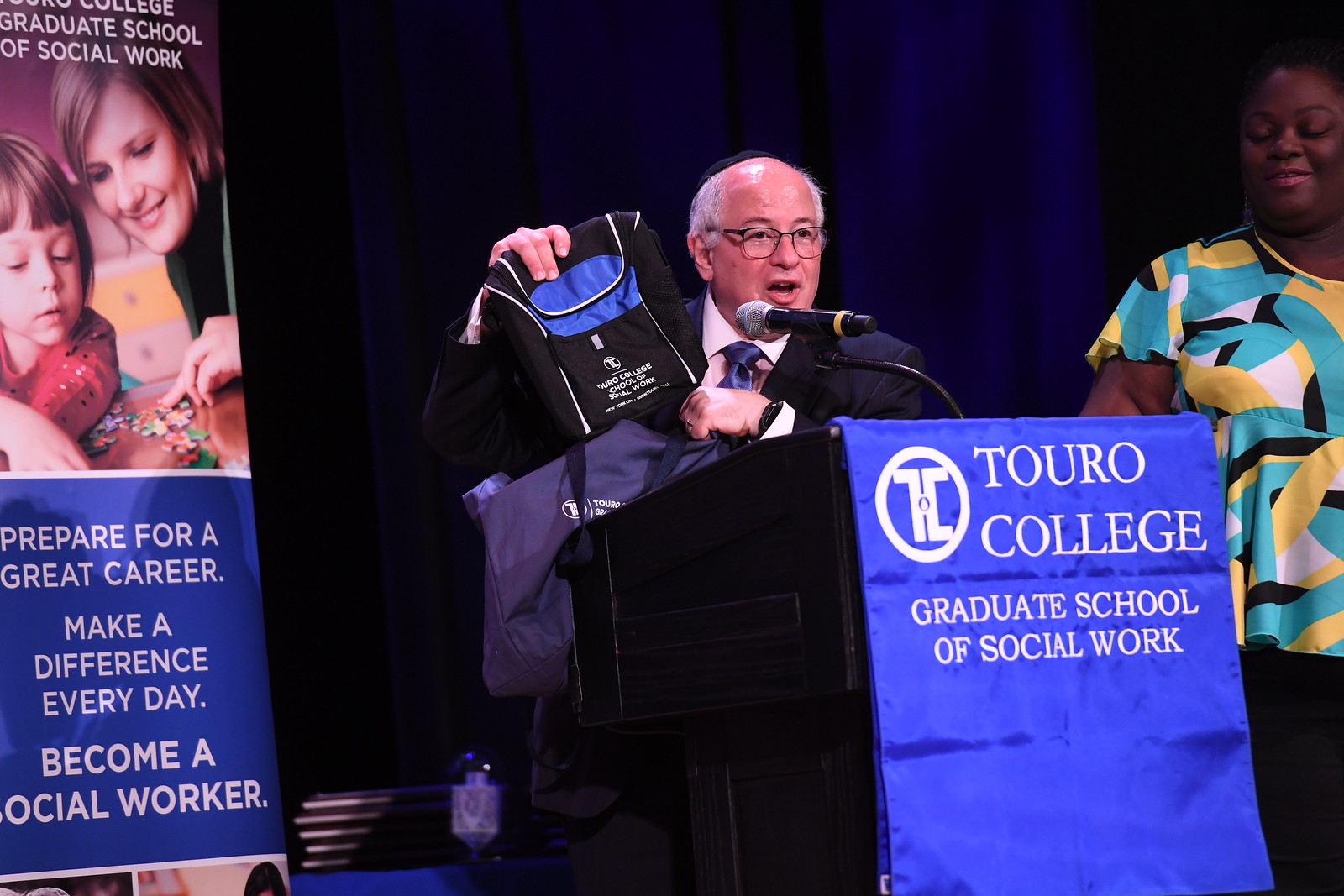In this detailed photograph taken in an indoor setting, a man is presenting behind a podium with a black background. The podium features a blue banner that reads "Touro College Graduate School of Social Work." The man, who has light skin, glasses, and is dressed in a black coat, white shirt, and blue tie, is speaking into a microphone attached to the podium. He is holding a black bag with a hint of blue and appears to be showing its contents. To his right, a woman with light skin and a warm smile is standing, wearing a colorful, patterned shirt with shades of green, yellow, black, and white. On the left side of the image, another banner can be seen depicting a woman and a girl playing with a puzzle, alongside text that reads "Prepare for a great career, make a difference every day, become a social worker." The background behind the man is mostly dark, with a blue curtain adding contrast.